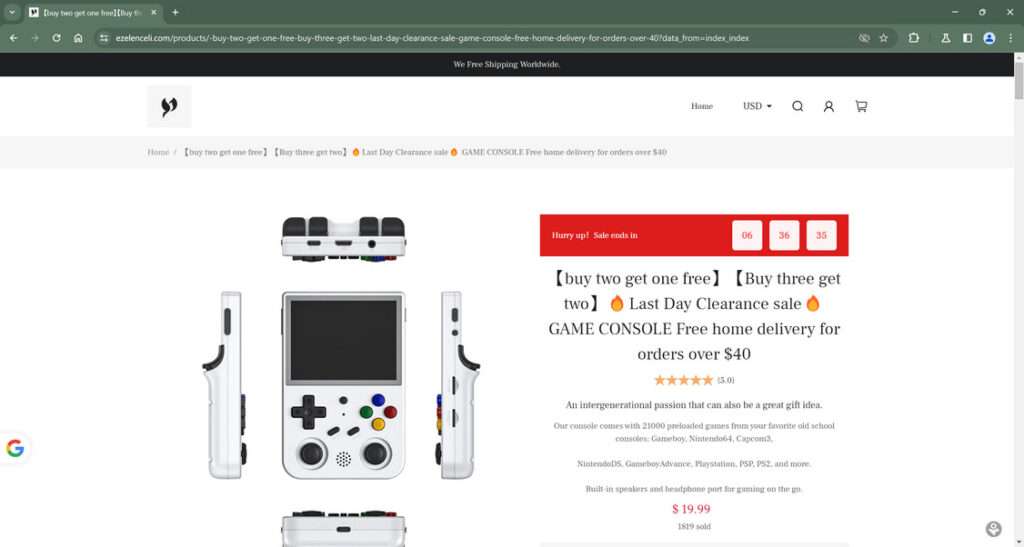A detailed screenshot of a web page displaying a white handheld gaming console reminiscent of a Game Boy. The web browser UI at the top features a sea green navigation and menu bars, which include an indistinct tab label and the typical minimize, maximize, and exit buttons. Beneath these are the browser buttons for back, forward, refresh, and other functions, followed by the URL bar, which contains an unreadable address. Next to the URL bar are icons for incognito mode, bookmarking, and various user profiles including a blue profile icon.

The web page itself has a black top bar with the text "FREE SHIPPING WORLDWIDE" in white. Below, on a white background, the Google 'G' icon in its characteristic red, yellow, green, and blue colors is situated at the bottom left. To the right, prominently displayed, is the handheld gaming console. The console is white with multi-colored buttons (green, blue, red, and yellow), gray D-pads, and circular pads. Further to the right, highlighted in the advertisement section, is text promoting a clearance sale with offers such as "Buy Two Get One Free" or "Buy Three Get Two," and a note on free home delivery for orders over $40.